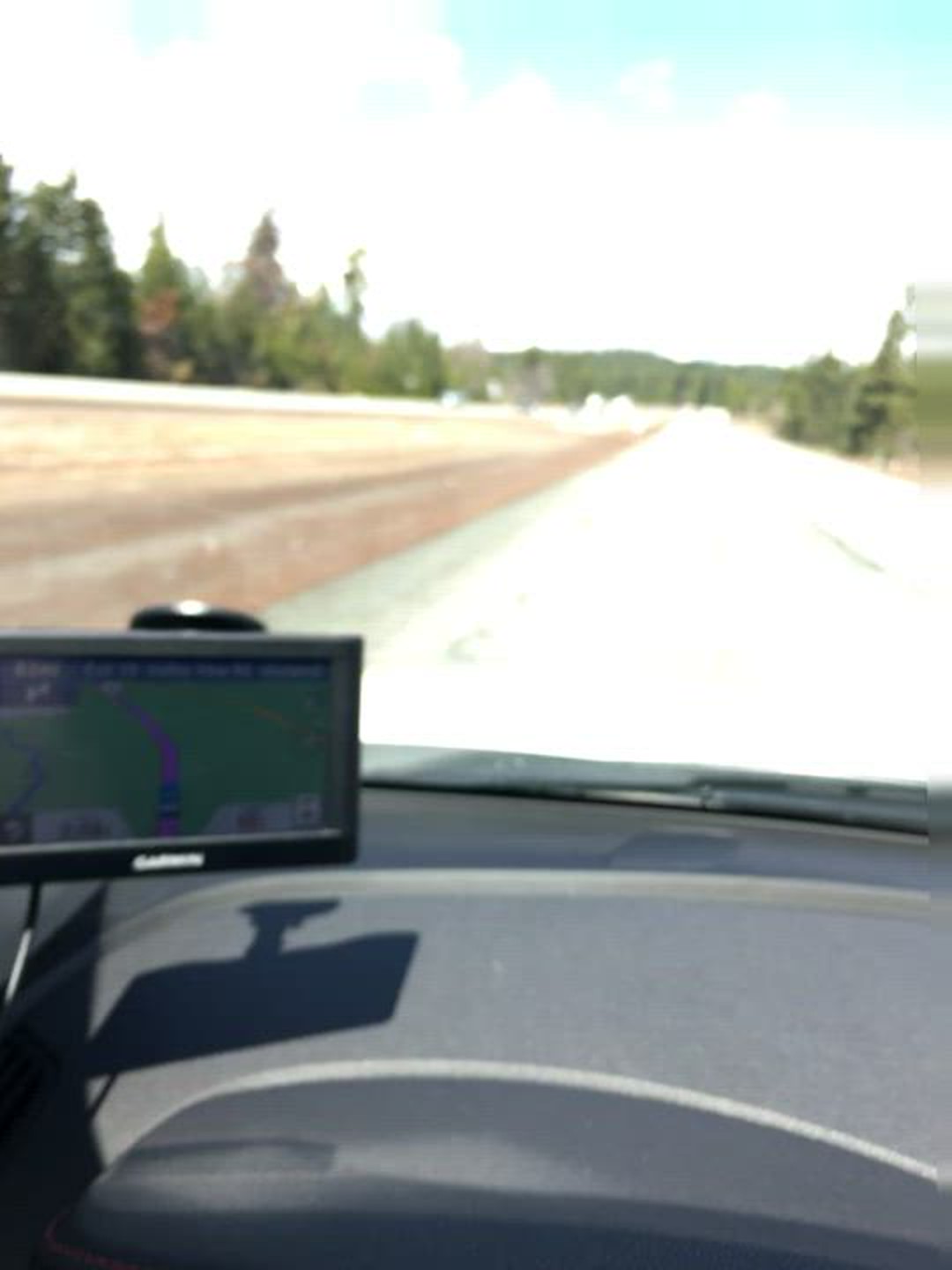A blurred, unsafe photograph appears to have been taken by the driver from within their moving vehicle, suggesting high speed. The image captures the dashboard and steering wheel in the foreground, emphasizing that the driver is behind the wheel. To the left, a GPS monitor displays navigational directions, indicating an active route. Through the windshield, a road flanked by trees on both sides stretches ahead, with what looks like a ditch visible on the left side of the road. The photograph's blurriness signifies motion, highlighting the potential danger of the driver snapping pictures while driving.